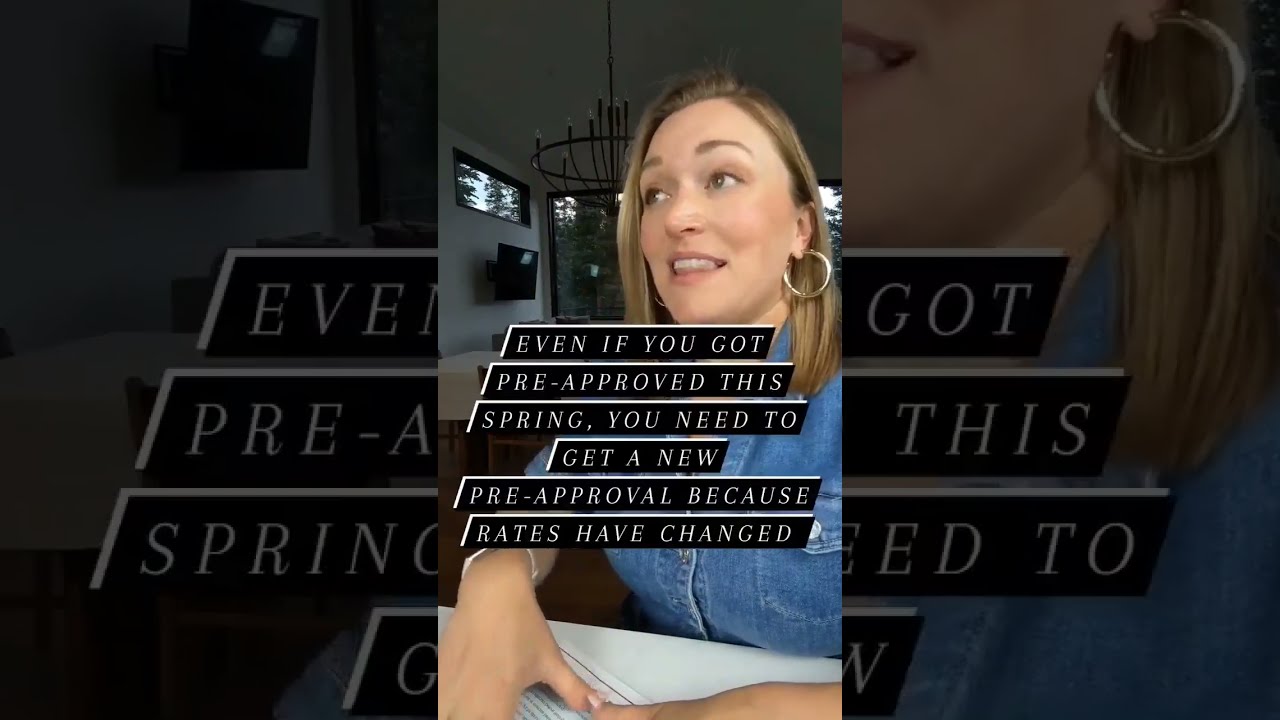In this image, we see a centered blonde woman, likely of Caucasian ethnicity with fair skin, sitting at a white table. She is dressed in a blue denim shirt and adorned with round gold hoop earrings, with pink-painted nails visible as her hands rest on the table. Her shoulder-length hair is parted to the left, with one side draping in front of her face and the other tucked behind her ear. The background reveals a well-lit indoor setting with white walls, a side wall to the right featuring a TV and a window, and additional windows to the left showcasing green trees outside. A chandelier is positioned above her, adding to the homey atmosphere. Overlaid text, in white letters on a black background with white drop shadows, spans the center of the image, stating: "Even if you got pre-approved this spring, you need to get a new pre-approval because rates have changed." This Instagram story or TikTok screenshot advises viewers on the necessity of obtaining new pre-approval due to changing rates. The overall colors in the image include white, black, blue, green, and hints of tan and gray.